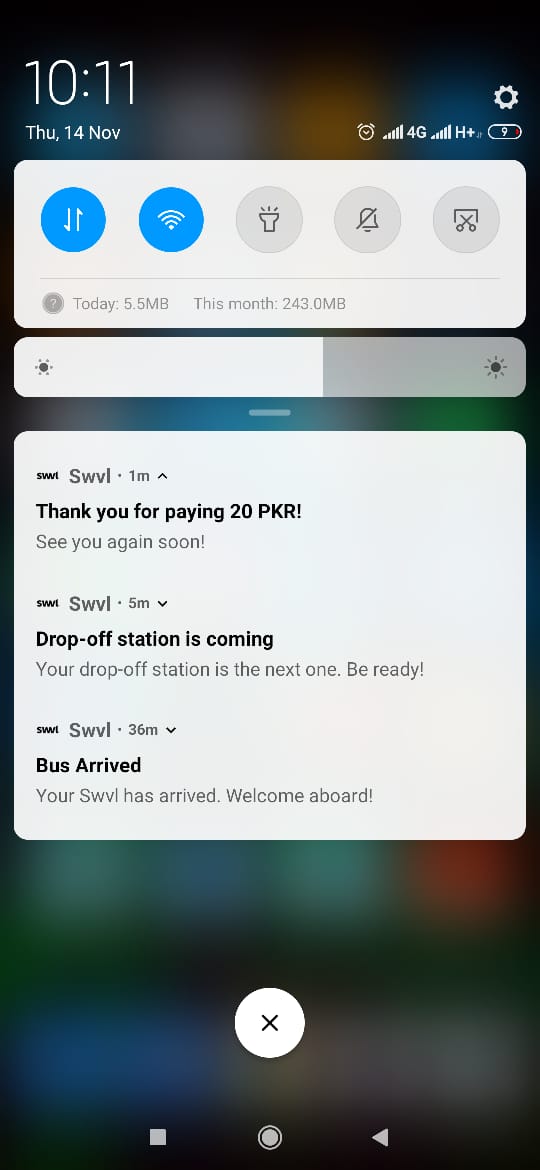The image showcases a smartphone screen displaying various elements prominently. At the top, the screen indicates the current time as 10:11 and the date as Thursday, 14th of November. The status bar includes icons for 4G connectivity, a clock, battery percentage, and Wi-Fi signal strength. Additionally, there are quick access icons for a flashlight, notifications, and a data usage tracker which indicates "Today: 5.5 MB" and "This month: 243 MB".

The brightness filter is visible, showing a range from the dimmest to the brightest setting, represented by a larger sun icon. Below the status bar, several notifications from the app SWVL are displayed. The first notification thanks the user for paying 20 PKR and wishes to see them again soon. The second notification, sent five minutes ago, informs the user that their drop-off station is approaching and they should be ready. The third notification, from 36 minutes ago, announces the arrival of the user's bus with a message welcoming them aboard.

At the bottom of the screen, an 'X' icon is present, likely for dismissing the notifications. The majority of the image features a white background with various text and screen settings contrasting against it.